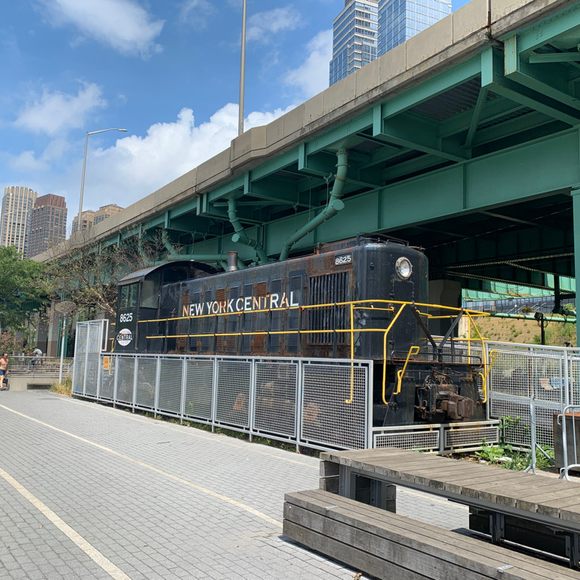The image depicts an outdoor scene featuring a prominently displayed, rust-covered, black train car with "New York Central" inscribed on its side in faded white lettering, along with the number 8625. The train car is encircled by light-colored metal fencing, and bright yellow railings contrast its aged appearance, indicating those parts have been freshly painted. Above the train, an overpass stretches diagonally from the middle left to the upper right, showcasing its aqua green metallic understructure. Surrounding the train are urban elements: on the left, there are towering skyscrapers against a blue sky adorned with scattered white clouds, and a cobblestone walkway with yellow stripes lies in the lower part of the image, suggesting a well-trafficked viewing area for passersby. The scene looks curated, possibly situated near a notable location like Central Park.